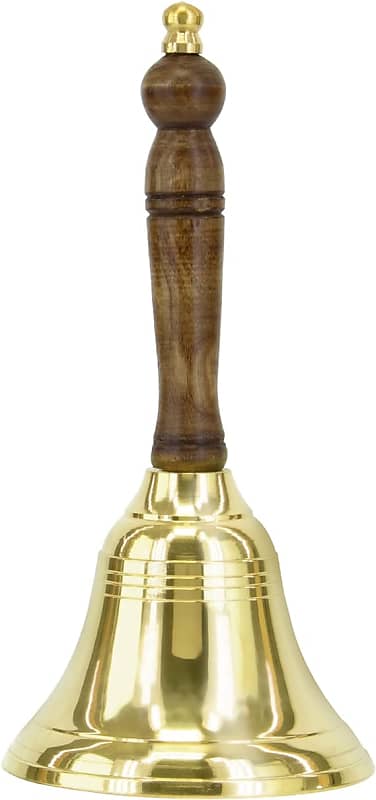The image is a detailed, full-color photograph of a shiny handheld bell, positioned upright with the handle facing upwards, centered against a pristine white background. The bell’s handle is made of polished brown wood, featuring a golden cap securely screwed into the base. The bell itself is golden and highly reflective, capturing a subtle reflection of the camera. Decorative circular cuts encircle the bell, with two circular cuts close to the top and one near the bottom. Additionally, there are vertical decorative lines on the golden bell; four lines adorn the upper portion, with two more further down. The photo emphasizes the bell as the primary focal point, showcasing its intricate design and reflective surface under presumably indoor lighting.